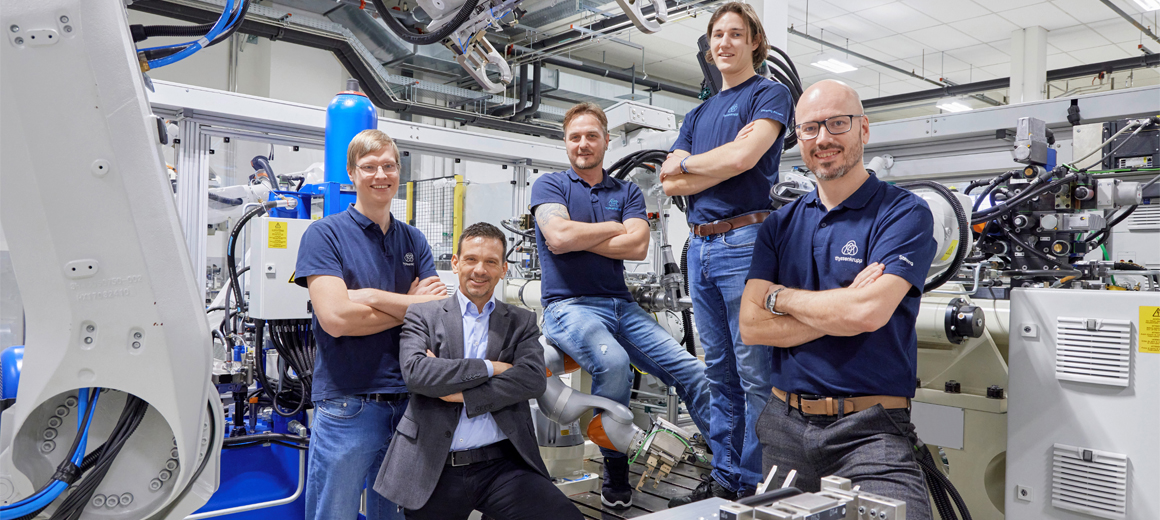In the image, five men are posed in a high-tech, machinery-filled room that closely resembles a laboratory or industrial cockpit. Most of the men are dressed similarly in blue polo shirts paired with jeans or denim pants. One man stands out in a charcoal gray sports jacket, light blue button-down shirt, and dress pants. All five have their arms crossed and are smiling, suggesting camaraderie and possibly indicating they are co-workers. The room is equipped with complex machinery, white wiring, and cream-colored equipment, giving an impression of a sophisticated, high-tech environment. Fluorescent lights illuminate the space, adding to the laboratory-like ambiance. Notably, the blue shirts worn by several of the men have a logo on the top right chest area, further hinting at a shared workplace or team identity.